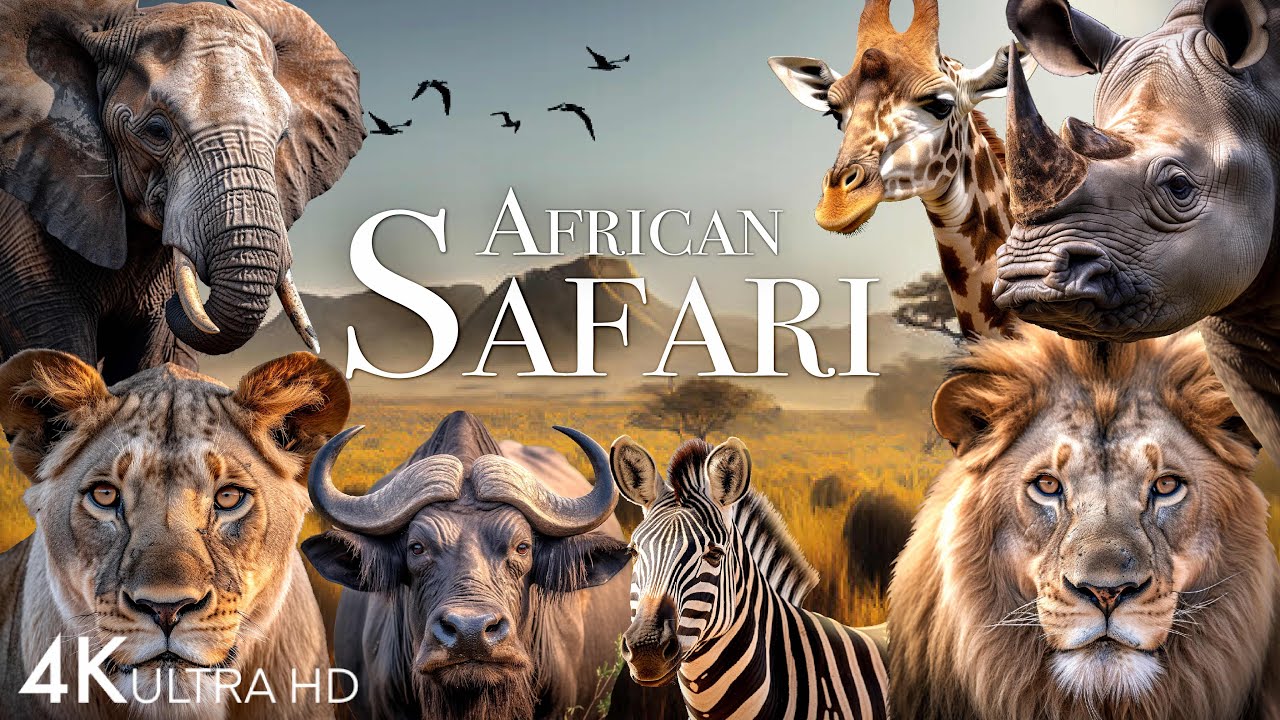This horizontal rectangular image appears to be a cover for a 4K Ultra HD video titled "African Safari." The title is prominently displayed in large white letters across the middle, with "African" above "Safari." The lower left corner also features the "4K Ultra HD" label. The cover showcases a vivid array of African wildlife, distributed across the image from the top left to the bottom left, then across the bottom, and up the right side. 

In the upper left corner is an elephant, while the bottom left features a lioness looking straight at the viewer, alongside what appears to be a water buffalo. Moving right across the bottom, there is a zebra and a male lion. The upper right section of the image hosts a rhinoceros with a giraffe positioned next to it. The background illustrates an African landscape, showing bare ground resembling a desert with some grassy areas and small trees in the middle. Further back, there are large hills or mountains, and the upper middle of the image features a light gray sky with several birds flying from left to right. The overall design seems to be a promotional edited shot for an African Safari video preview.